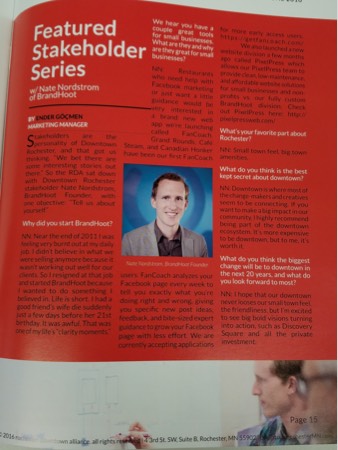**Detailed Caption:**
This vivid, full-color photograph captures the right-hand page of a physical magazine. The page is predominantly covered in a striking red background, occupying approximately the top four-fifths of the layout. Against this bold red backdrop, the article titled "Featured Stakeholder Series with Nate Nordstrom of Brand Hoot" is showcased. 

The text within the article is a sophisticated blend of black paragraphs and interspersed white headings, creating a visually engaging contrast. Though the specific content of the article remains indistinct in the photograph, the headings hint at an interview format with questions and responses, addressing topics such as "Why did you start Brand Hoot?" and "What's your favorite part about Rochester?"

The bottom fifth of the page transitions to a clean white background, featuring an image of a man intently drawing with a marker on a whiteboard, adding a dynamic visual element to the overall design. The layout and color choices combine to craft an aesthetically appealing and informative magazine page, highlighting Nate Nordstrom's insights and experiences with Brand Hoot.